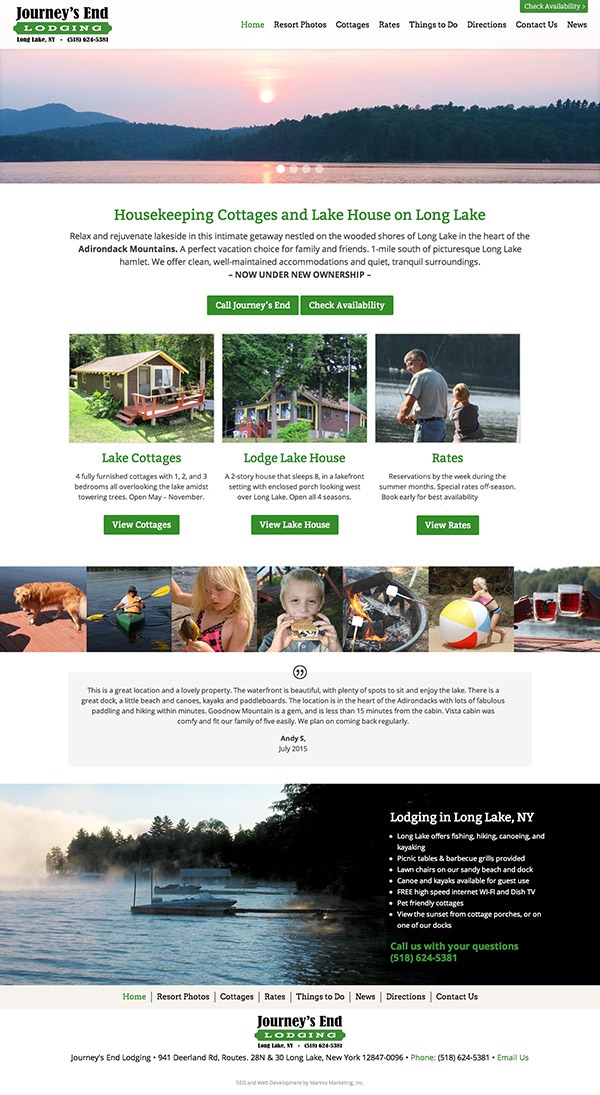The webpage features a serene and inviting design for Journey's End, a lodging destination located in Long Lake, New York. At the top, the site title "Journey's End" is prominently displayed in black text against a white background. Directly below is a green banner with white text that reads "Lodging," followed by the location "Long Lake, New York" and a reference number "(518) 625-381," likely for contact purposes.

On the right side of the page, a navigation menu allows visitors to explore various sections: Home, Resort Photos, Cottages, Rates, Things to Do, Directions, Contact Us, and News. Below the navigation, another green banner in white text invites visitors to "Check Availability."

The webpage showcases a stunning outdoor banner depicting beautiful natural scenery, including the sky, sun, mountains, trees, and water—offering a glimpse into the picturesque environment of Journey's End.

Further down, there's a section with a white background and green text detailing the "Housekeeping Cottages and Lake House on Long Lake." This portion provides descriptive information about the accommodations available, noting that the property is now under new ownership and encouraging visitors to contact Journey's End for more details. A green tab with white lettering again prompts users to "Check Availability."

The site highlights three specific accommodation options: Lake Cottages, Lodge Lake House, and their respective rates. Visitors have the opportunity to view images and details of each option. Additional photos show guests engaging in various activities available at the location.

Towards the end of the page, a review section offers testimonials, followed by another banner emphasizing outdoor activities and lodging options at Long Lake. Bullet points provide essential contact information, and a footer mirrors the top navigation menu, making it easy for users to find Home, Resort Photos, Cottages, Rates, Things to Do, News, Directions, and Contact Us.